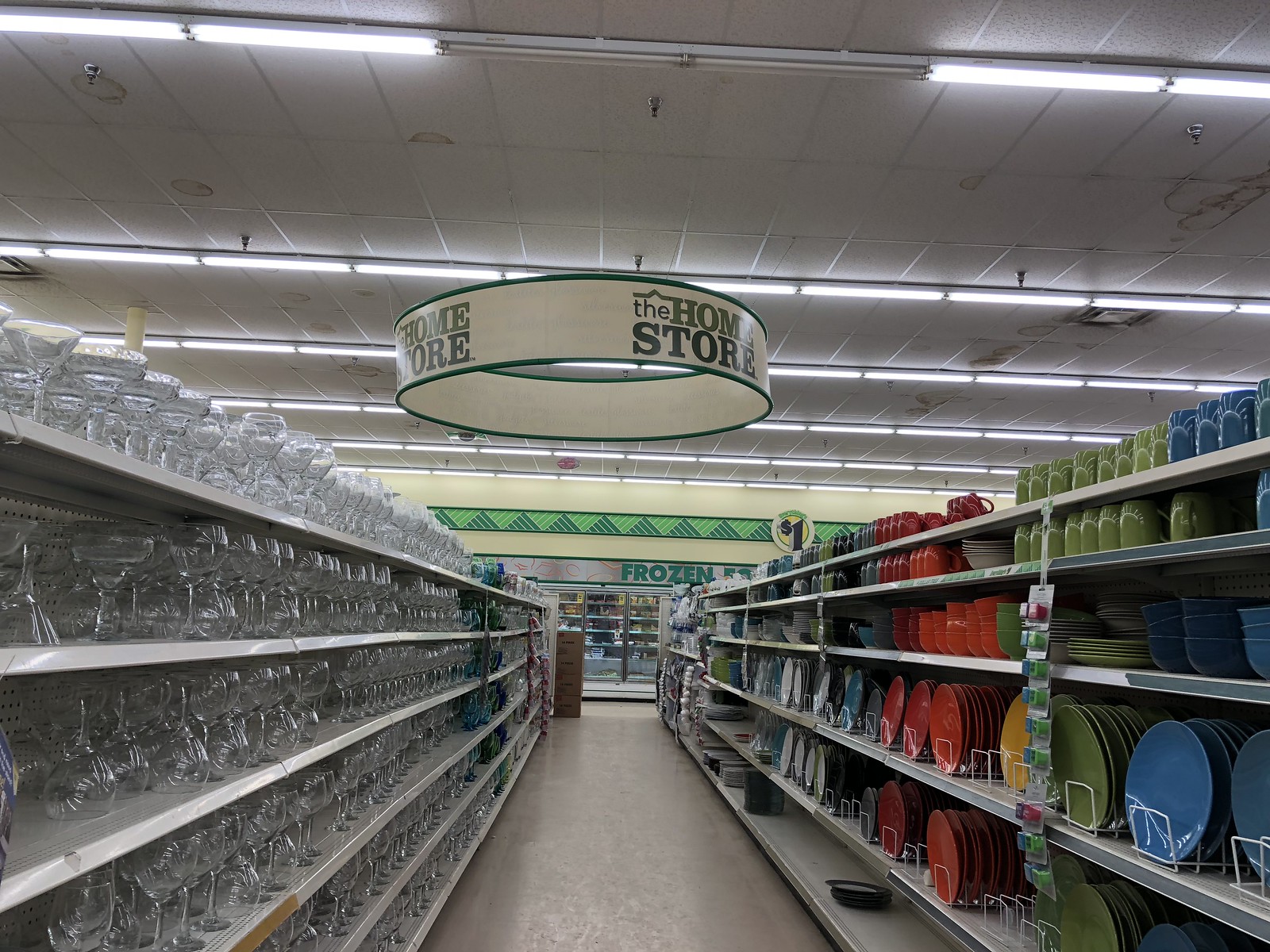This photograph captures a detailed view inside a large store aisle, potentially a dollar store, identified by a small circular sign on the back wall that indicates "one dollar" in black text with a yellow center. The aisle is flanked by six shelves on either side, displaying an array of glassware and crockery.

On the left side, the shelves are filled with varied glassware, predominantly clear goblets in different shapes and sizes, with blue and green glass items appearing further down the aisle. Conversely, the right side features assorted crockery organized by color. The top two shelves display vases or jug-like containers, followed by bowls and plates on the subsequent shelves. Plates have been slotted upright in racks on the next two shelves, with the bottom shelf nearly empty, containing some undistinguishable containers. The color arrangement of the plates starts with blue at the front and transitions to green, yellow, orange, red, gray, teal, white, and black as they proceed down the aisle.

Suspended from the ceiling is a circular banner bordered with dark green edges and the phrase "The Home Store" written in green text, indicating the section of the store. The ceiling also features rows of fluorescent lights, visible water sprinklers for fire safety, and blotchy marks suggestive of water leaks. In the background, the end of the aisle is marked by a frozen food section with glass doors and stacked cardboard boxes.

This richly detailed scene embodies the organized yet cluttered charm of a budget-friendly home goods aisle.